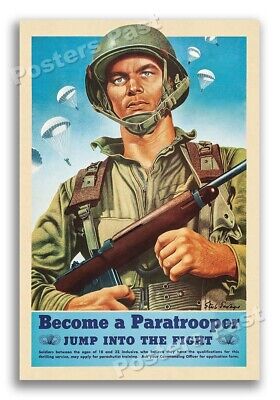The image is a vintage World War II propaganda poster with a distinct watermark reading "Posters Past" on the top left and bottom right corners. The main subject of the poster is a drawn, attractive Caucasian soldier dressed in green army attire, including a helmet with a chin strap secured tightly. He is carrying an M1 carbine rifle and appears to be wearing a parachute backpack. The soldier is depicted with a serious expression and hazel eyes. Behind him, the background features a blue sky with white clouds and paratroopers descending with open parachutes. At the bottom of the poster, in bold dark blue letters against a baby blue background, are the words, "Become a Paratrooper. Jump into the fight." Additional, smaller text is also present but is too small to read clearly. The overall impression of the poster is very heroic and patriotic, typical of wartime propaganda.